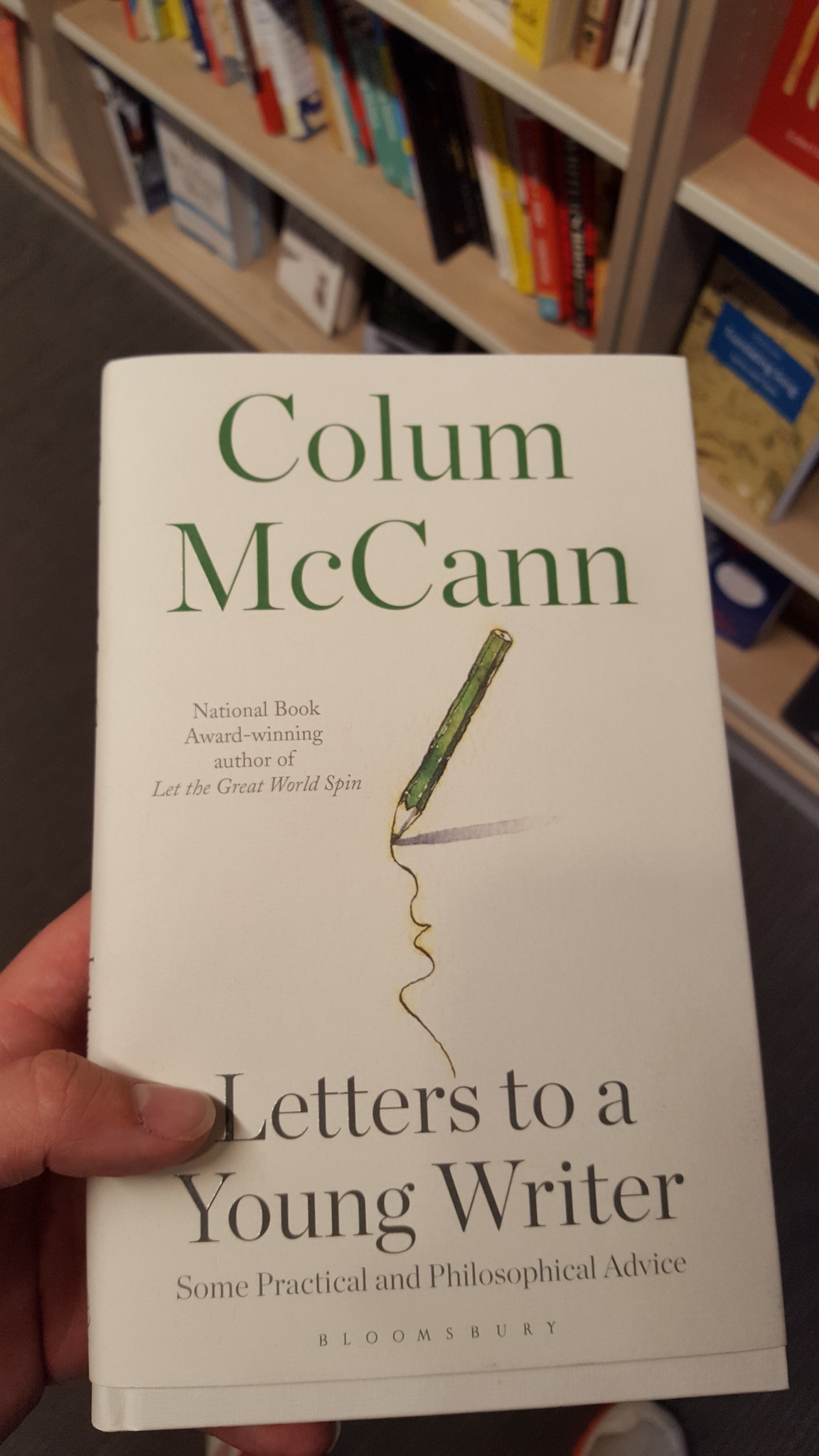The image depicts a top-down view of a person standing and holding a book with their left hand, their thumb resting near the spine. The environment appears to be a library or bookstore, as evidenced by the bookshelves visible in the background.

The book has a white cover with minimalist design elements. At the top, in green font, it prominently displays the author’s name, "Colum McCann," who is noted as the "National Book Award-winning author of Let the Great World Spin" in smaller, darker text beneath. The title, "Letters to a Young Writer," is accompanied by the subtitle "Some Practical and Philosophical Advice." The publisher, Bloomsbury, is also mentioned on the cover.

An illustration of a pencil with a watercolor effect and a curved line further embellishes the cover. Visible beneath the book are the person's feet, reinforcing that the photo is taken from above.